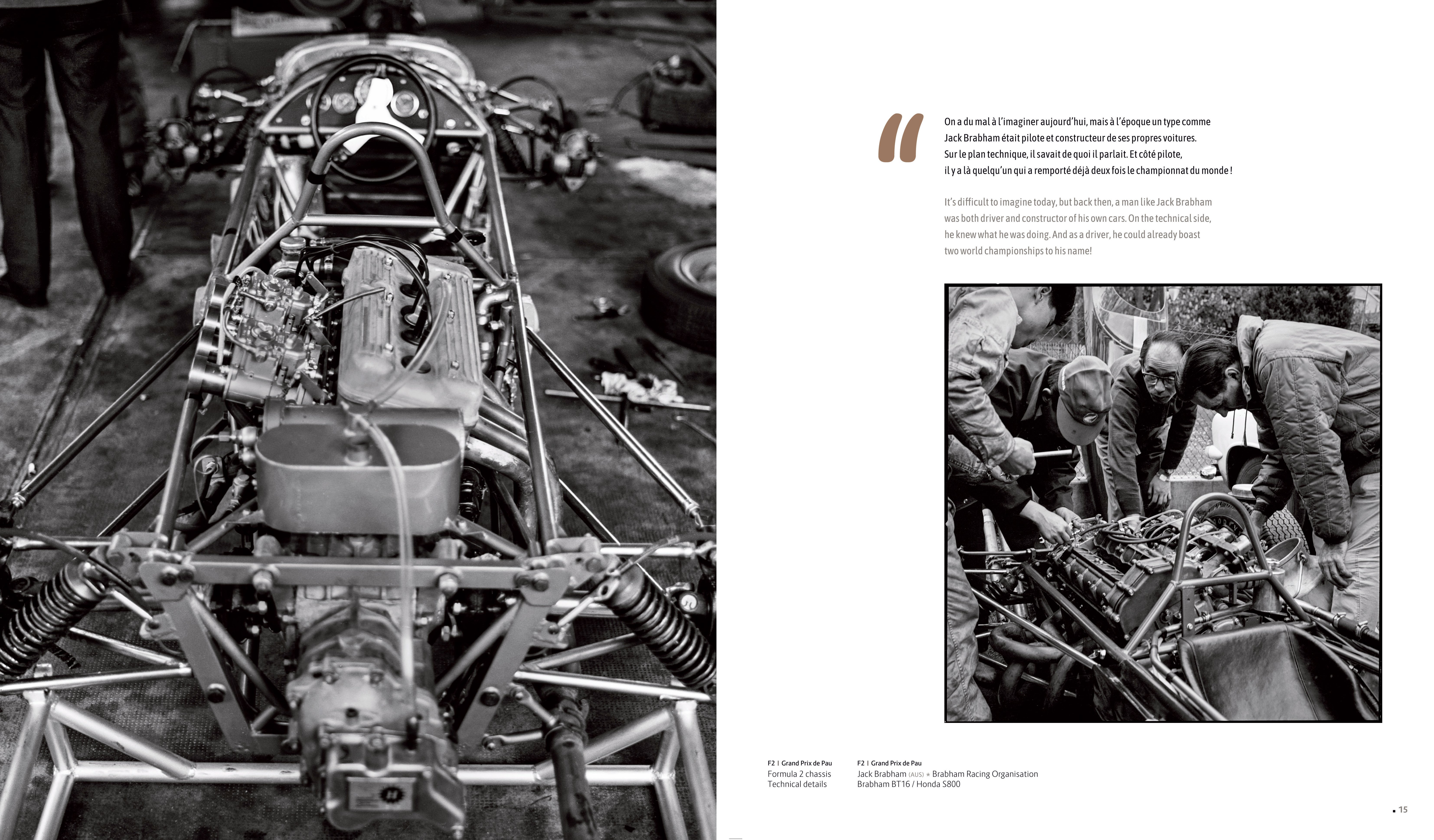The image consists of two black-and-white photographs. The larger photo on the left showcases the stripped-down framework of a race car, possibly featuring a four-cylinder engine, a single-person driving compartment, and visible components such as the engine block, steering wheel, and shock absorbers. This contraption appears metallic and skeletal, resembling a structural device. On the right, a smaller square photograph displays four individuals attentively working on the same race car's engine. The individuals, dressed in varied attire including a puffy jacket, long-sleeved shirts, and a cap, are huddled around the engine, engrossed in adjustments or discussions. Accompanying this image, there is a white page with black text, including a note mentioning Jack Robham as both driver and constructor of his cars, underscoring his dual achievements in both engineering and racing, having secured two world championships.